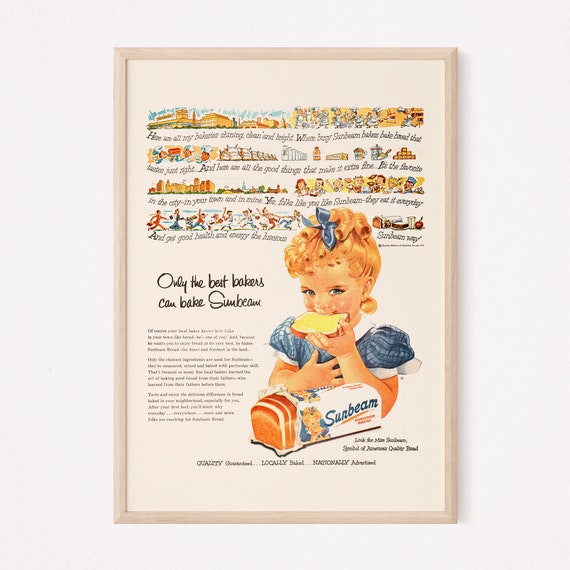This detailed and descriptive caption for the image combines shared elements and unique details from both descriptions for a comprehensive summary.

---

The image features an advertisement, framed in a light tan wooden rectangular frame, showcasing a delightful illustration or painting of a young girl, approximately seven or eight years old. She has white, rosy skin and her hair is tied up in a bun, adorned with a blue ribbon. The girl is depicted wearing a short-sleeve blue top with a white collar and white trim on the sleeves. In the picture, she is using her left hand to hold up and eat a piece of bread, with a loaf of bread placed in front of her. The loaf, wrapped in white packaging, prominently displays the brand name "Sunbeam" in blue. Additionally, the advertisement includes text that reads, "Only the best bakers can bake Sunbeam quality guaranteed locally baked nationally advertised," along with smaller images along the top that illustrate the bread-making process. The girl herself is also drawn on the bread wrapper, creating a cohesive and charming promotional piece.